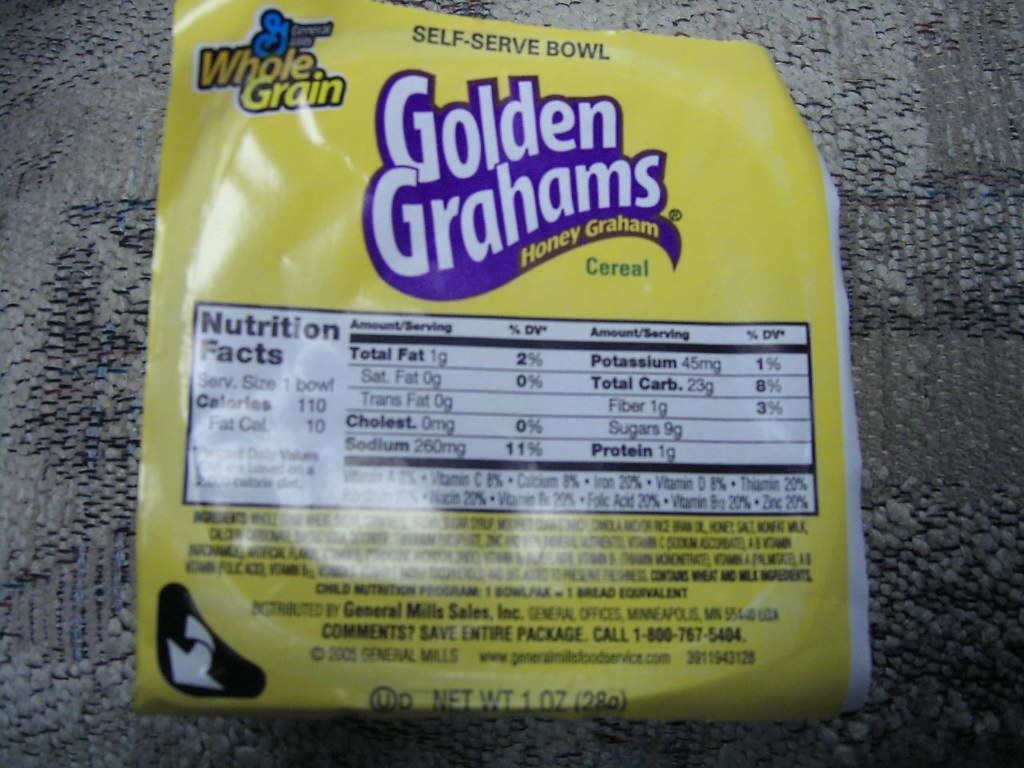The image showcases a piece of carpet, upon which rests a package, specifically a self-serve bowl of cereal by General Mills. The packaging highlights the nutritional content of the Golden Grahams Honey Graham variety. The product name "Golden Grahams" is prominently displayed in bold white letters within a striking blue ribbon, while "Honey Graham" is highlighted in yellow letters within the same ribbon. The packaging also includes essential nutritional information: 1 gram of total fat, 0 grams of trans fat, 0 milligrams of cholesterol, and 260 milligrams of sodium (11% of the daily value). Additionally, it lists 45 milligrams of potassium (1% of daily value), 23 grams of total carbohydrates (8% of daily value), including 1 gram of dietary fiber (3% of daily value) and 9 grams of sugars. The cereal also contains 1 gram of protein.